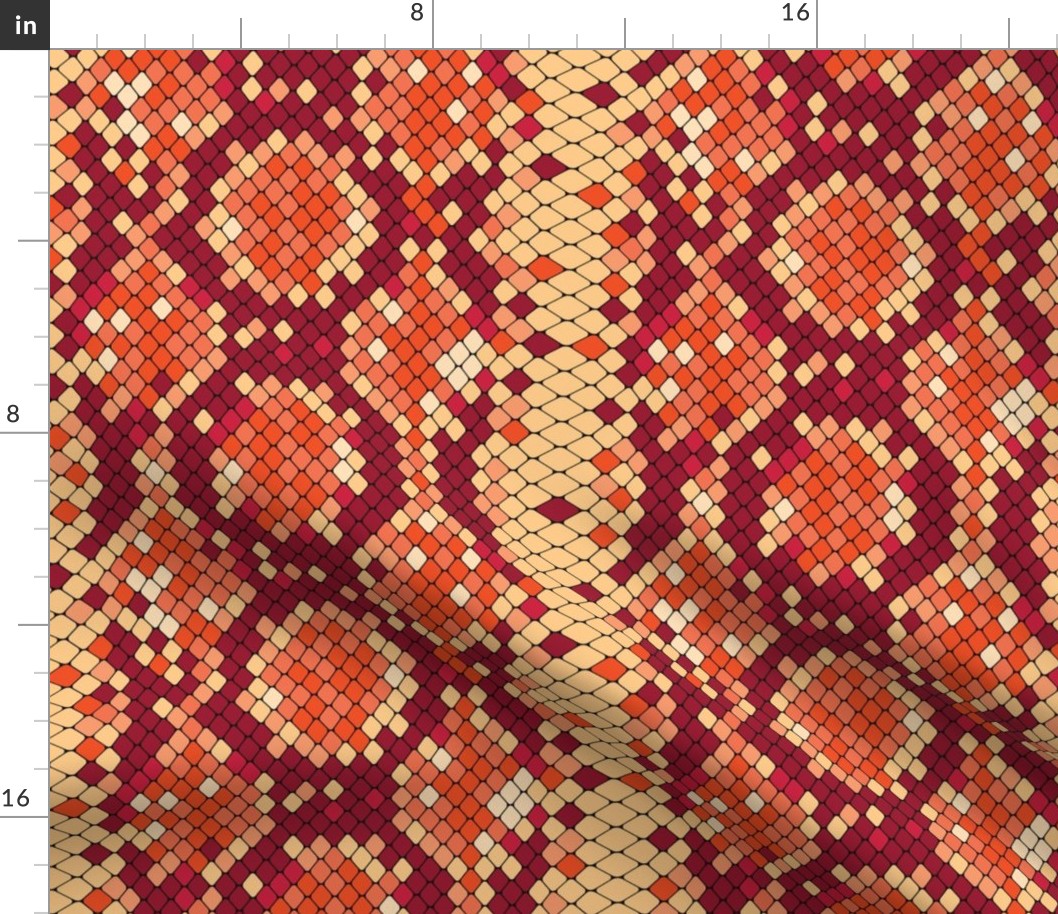The image depicts a large square piece of fabric with a complex, colorful pattern. The fabric features a mosaic-like array of overlapping diamond shapes, made up of tiny individual diamonds. The primary colors woven into the fabric are light tan, white, red, orange, and cream, with these hues blending to form an intricate, vibrant design somewhat reminiscent of snake skin. The pattern has distinctive orange and yellow variations, punctuated by light brown diamond shapes, particularly in a central strand that divides the design. Surrounding these shapes is a red background, enhancing the contrast and depth of the central motif.

The left side and the top edge of the image are bordered by a ruler scale marked in inches, with numbers clearly displayed at intervals—8, 16, and so on—indicating precise measurements. The top corner of the image includes a small black box with white writing that reads "in," further affirming the measurement indication. The fabric's pliability is evident from two prominent folds visible at the bottom center, emphasizing its texture and volume.